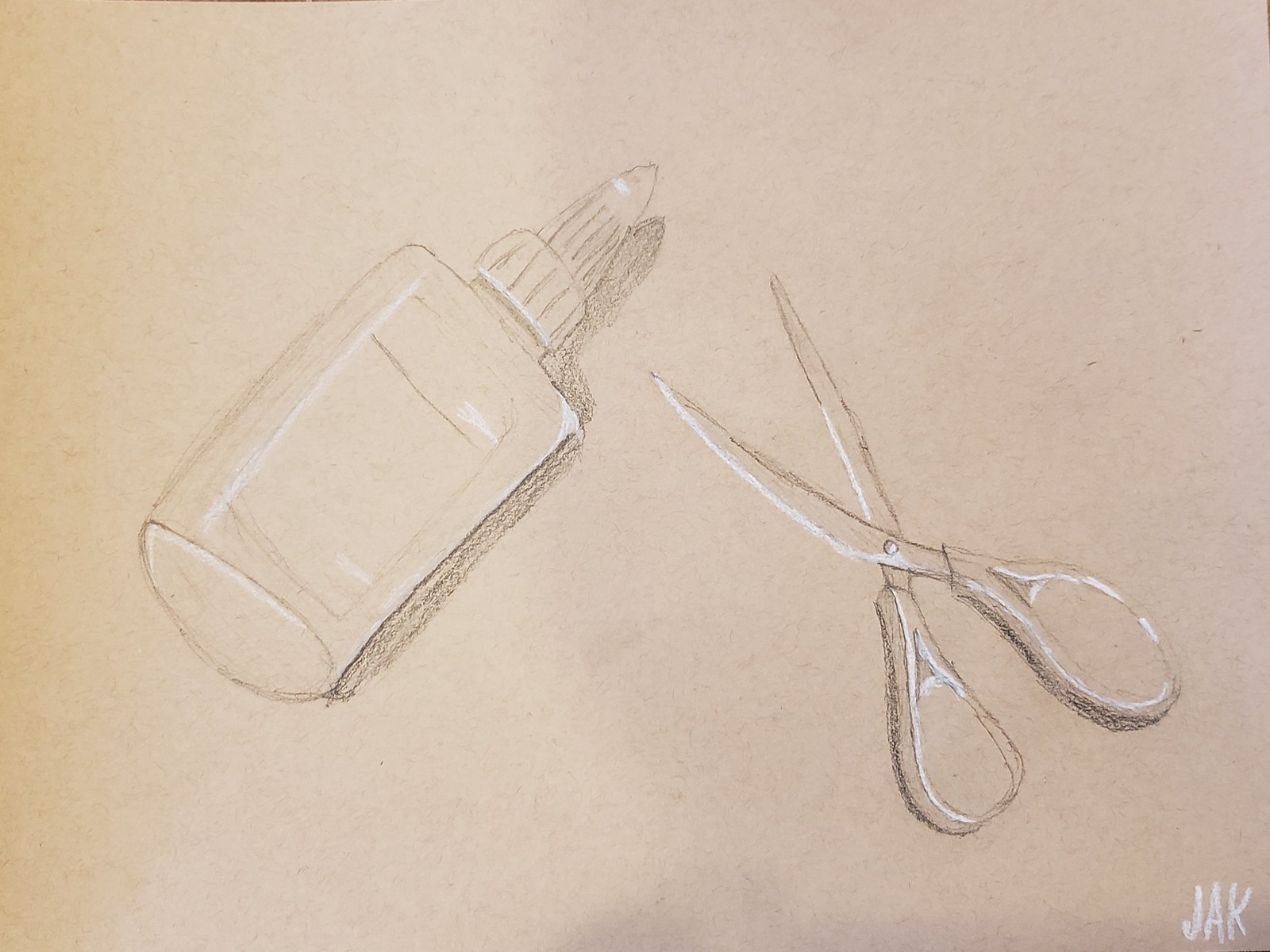The image presents a detailed pencil drawing on a tan, nearly square piece of paper, possibly resembling parchment or craft paper. The composition features a bottle of glue—likely resembling Elmer's glue—lying on its side on the left side of the paper and outlined in black pencil with white shading for depth. The glue bottle, characterized by a short, wide neck and a twist cap with vertical pencil lines, casts a subtle shadow to its right. Positioned on the right side and angled towards the left, a pair of scissors with partially open blades are depicted, with their handles facing down and blades facing up. The scissors are similarly outlined in black pencil with white detailing along the handles and blades. The drawing's lower right corner is marked with the artist’s initials, "J.A.K.," printed in capital letters.